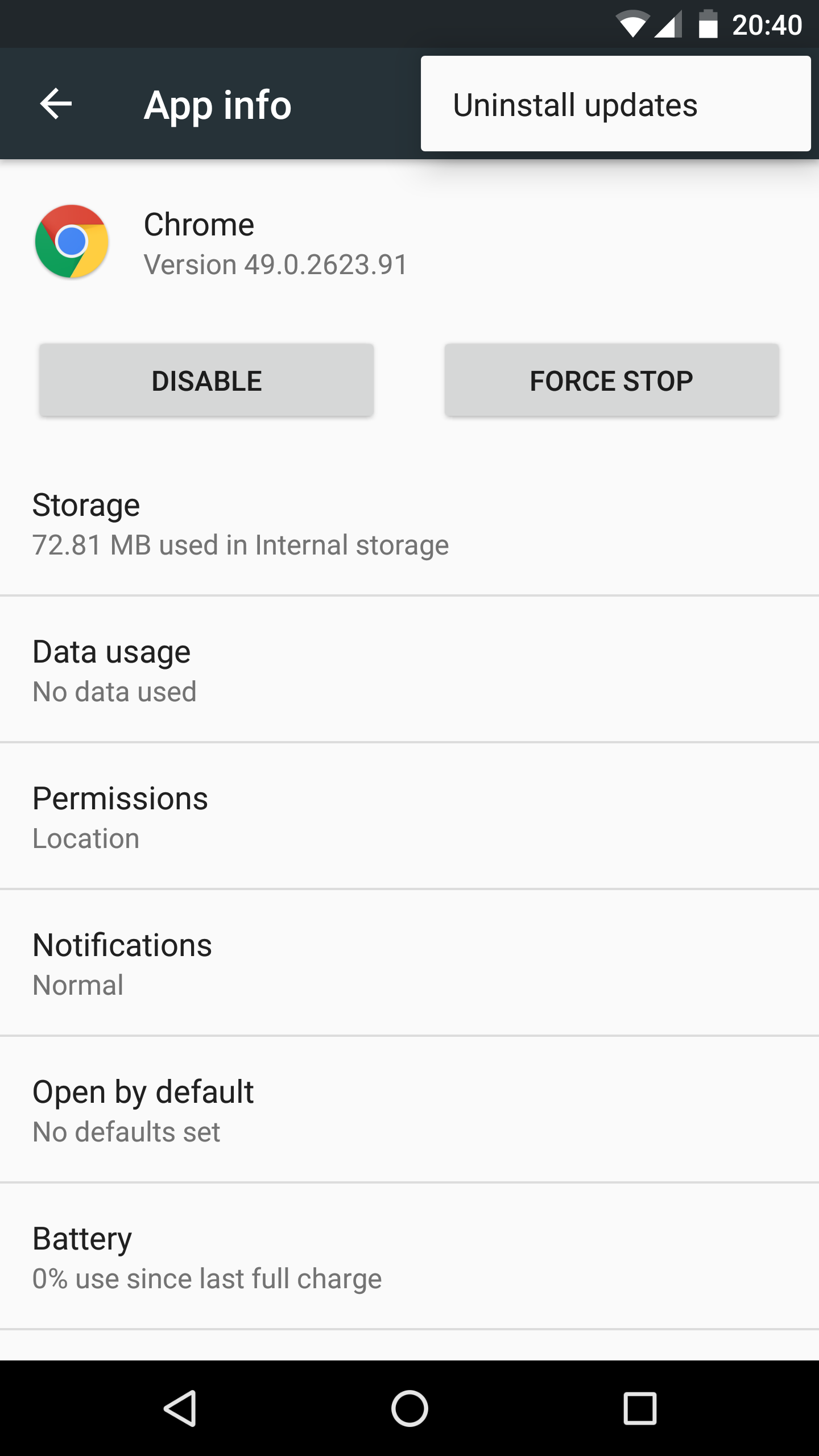This detailed image depicts a screenshot of an application information page for Google Chrome on an Android device. The header at the top of the screen is black, with white, bold text on the left that reads "App info" alongside a left-pointing arrow. In the upper-right corner, there are icons representing Wi-Fi reception, battery life, and the current time, which reads 20:40.

Just beneath the header, a prominent white button with black text labeled "Uninstall updates" is visible. The main section of the page features the Chrome icon next to the word "Chrome" and the version number 49.0.2623.91.

Further down are two gray action buttons; the left button labeled "Disable" and the right button labeled "Force stop." Below these buttons, additional information about the app is provided on a white background in black text, including:
- Storage: 72.81 MB used in internal storage.
- Data usage: No data used.
- Permissions, notifications, open by default, and battery.